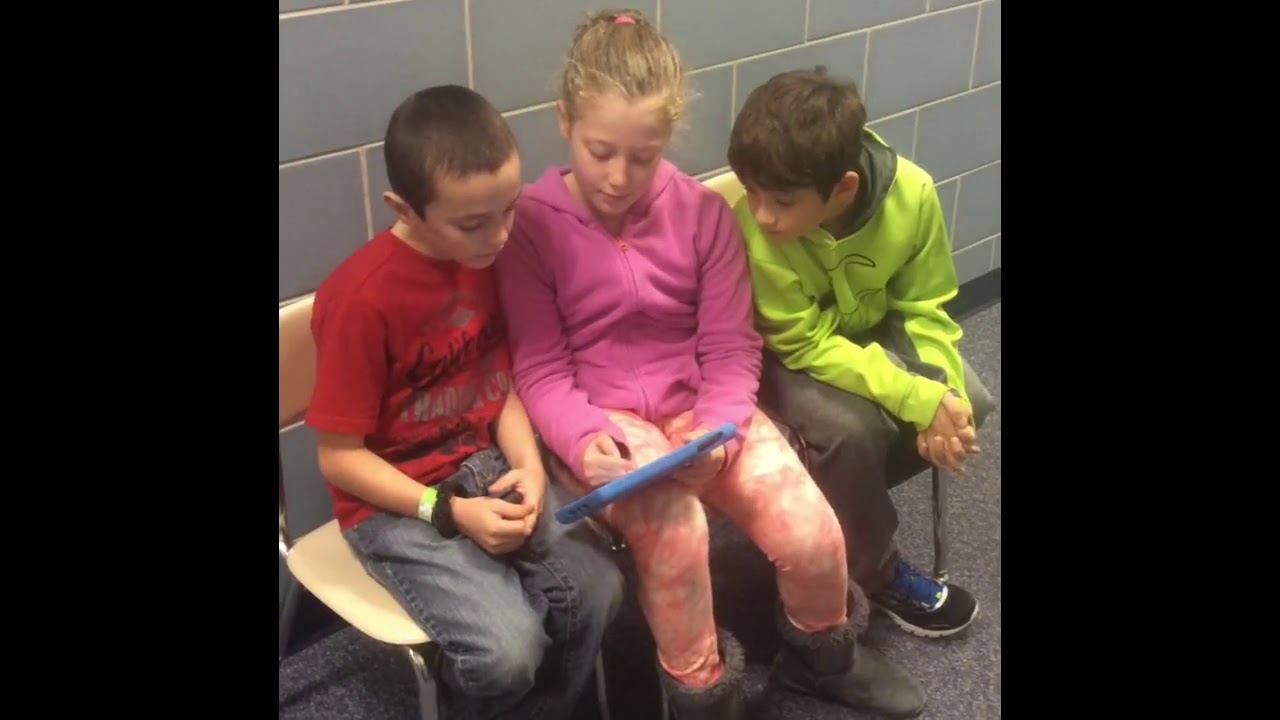In this photograph, captured indoors, likely in a school hallway, three children are closely seated together on a beige bench against a teal-colored brick-tile wall. The children, appearing to be between the ages of 8 and 12, are arranged with a girl in the middle and two boys on either side. The boy on the left wears a red t-shirt, blue jeans, and a bracelet on his right arm, with a close-shaved head. The girl in the middle sports a pink sweater, salmon-colored leggings, and black boots, her blondish hair pulled back with a pink scrunchie. She holds a tablet encased in blue, showing and pointing at something on the screen, which both boys are attentively observing. The boy on the right, with short brown hair, is dressed in a green sweater, black jeans, and tennis shoes. The overall image, possessing a horizontal rectangular form, features enough detail to capture their engaged expressions and the vibrant, varied colors of their attire.